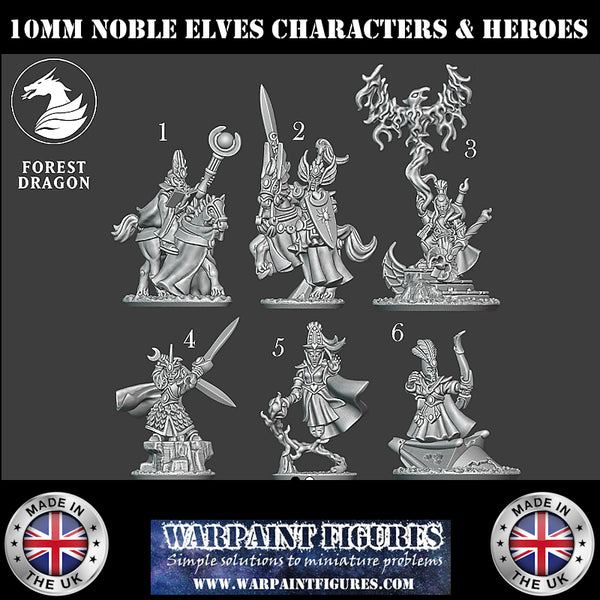The image is an advertisement showcasing six detailed 10mm Noble Elves action figures, depicted as characters and heroes. At the top of the image, bold text reads "10mm Noble Elves, Characters and Heroes," against a grey background. Accompanying this title is a logo featuring a dragon and the text "Forest Dragon." Each figure is unique: some Elves ride horses brandishing swords, staves, or bows, and one elf holds onto a dragon's tail. The bottom of the image features a broad black bar with the Warpaint Figures logo and their slogan "Simple Solutions to Miniature Problems" alongside the website "www.warpaintfigures.com," all set against a night sky filled with stars. Two British flags, resembling medallions, are positioned at the bottom left and right corners, indicating the figures are made in the UK. This enticing display suggests that the figures are intended for painting and use in various crafts or games.